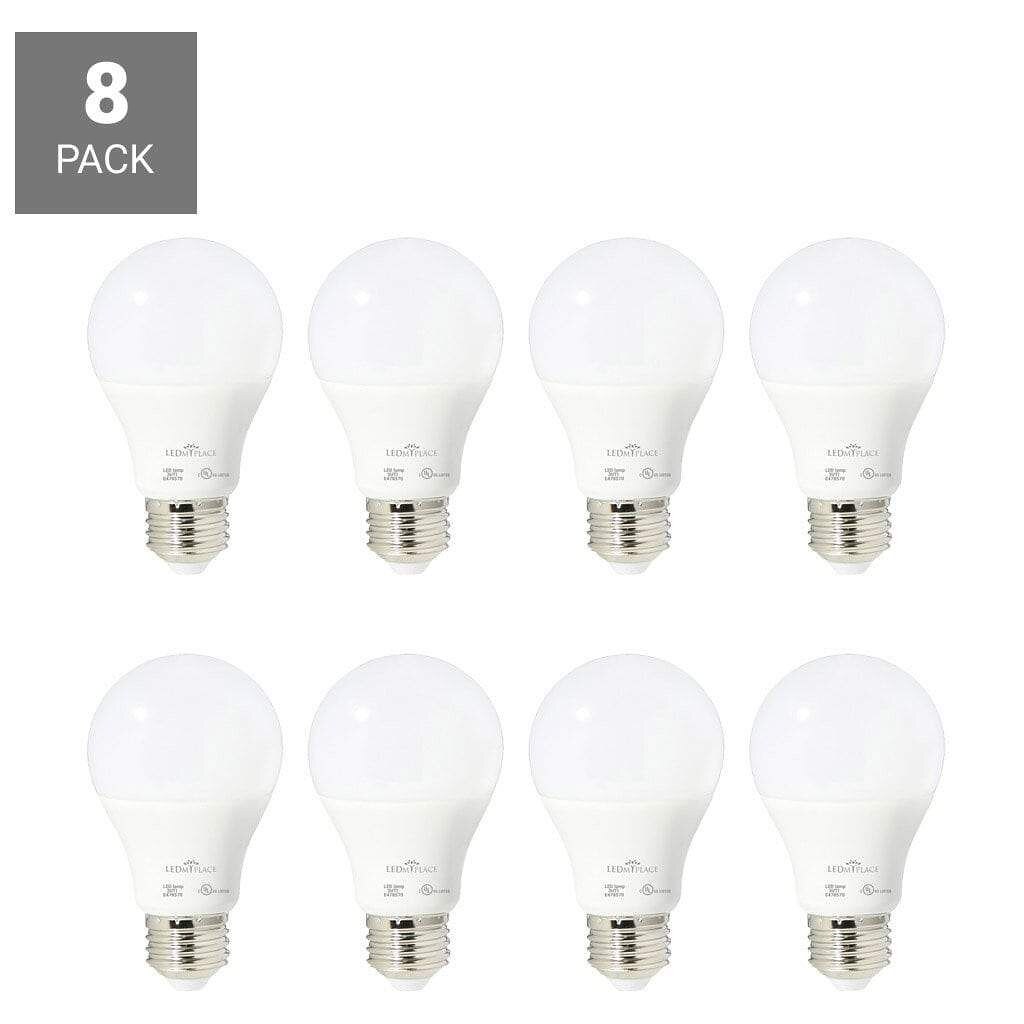The image displays eight traditional-looking light bulbs arranged in two neat rows of four each on a plain white background. Each light bulb is medium in size with a white glass bulb at the top and a silver screw base at the bottom. The bulbs feature some small, unreadable gray writing on a slightly darker white plastic portion just above the screw base. In the upper left corner of the image, a gray box with bold white text reads "Eight Pack," giving the impression that the bulbs form part of a packaged eight-pack set, although no actual box is shown in the image. The light bulbs are all new and identical in appearance, exhibiting a classic design that has been in use for years.